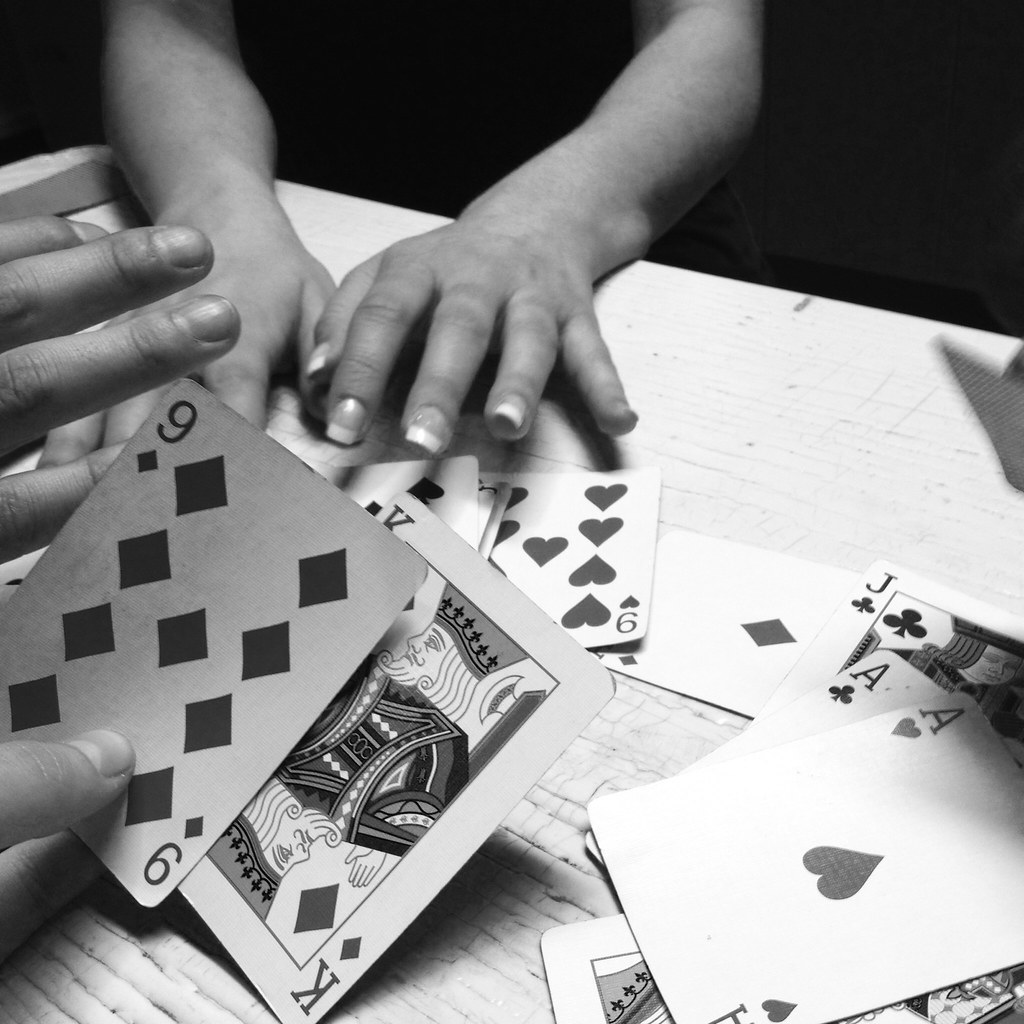In this evocative black-and-white photograph, the scene is tightly focused on a small, light-colored table where an intense card game is unfolding. The close crop brings attention to the hands of the players, emerging from the shadows that envelop the background. The hand in the foreground, reaching from the bottom left corner, clutches a nine of diamonds and a king of diamonds, the meticulously detailed French tip manicure hinting at the player's composed demeanor. Scattered across the narrow table are various cards including the ace of hearts, ace of clubs, jack of clubs, a barely identifiable diamond card, a queen, a nine of hearts, and a spade that remains partially concealed. The stark contrast between the bright table and the deep darkness surrounding the players' hands creates a dramatic and mysterious atmosphere, drawing the viewer into the suspense of the game.